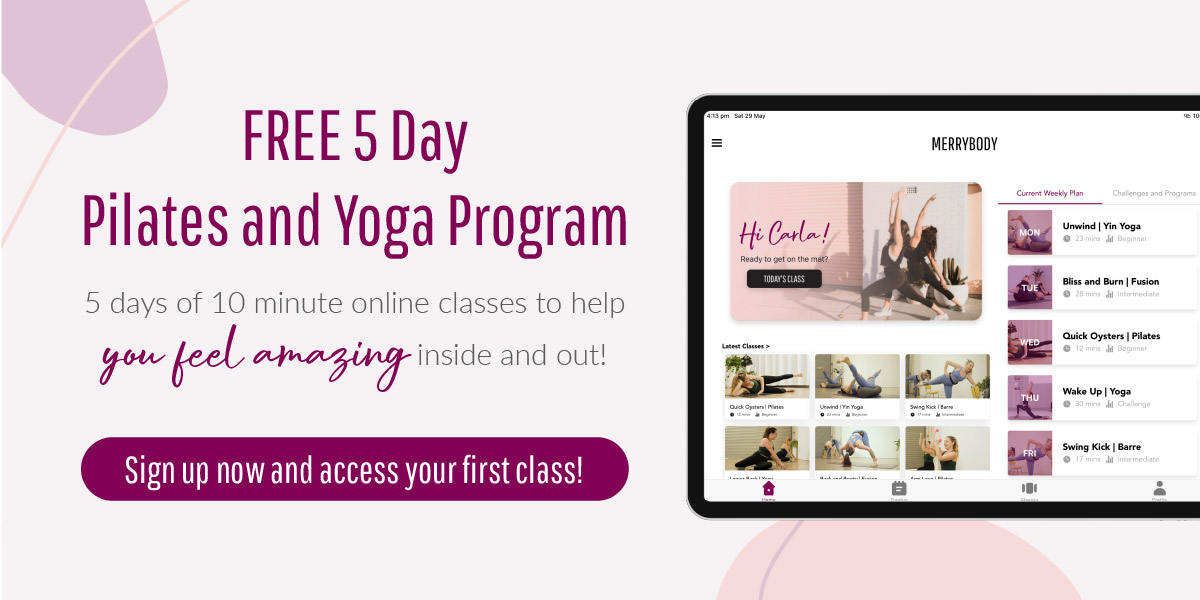The background of the image is a gradient blend of gray and purplish hues, darker at the top. In the foreground, there is a prominent shape reminiscent of the end of a thumb, featuring a curved tan line. Below this shape, the text "Free 5 Day Pilates and Yoga Program" is displayed in purple. Underneath that, a smaller text in a sans-serif font reads, "5 Days of 10 Minute Online Classes to Help You Feel Amazing Inside and Out," with "You Feel Amazing" highlighted in purple cursive. A large purple button is located below this message, containing white text that instructs, "Sign Up Now and Access Your First Class."

On the right side of the image, a simulated screen display appears with a black border. The screen shows a webpage with a white background. At the top center of the webpage, the text "Merry Body" is displayed. Below this header, a large picture depicts individuals practicing yoga. The greeting "Hi Carla" is visible, followed by a black button beneath the image. The text on the button is too small to discern.